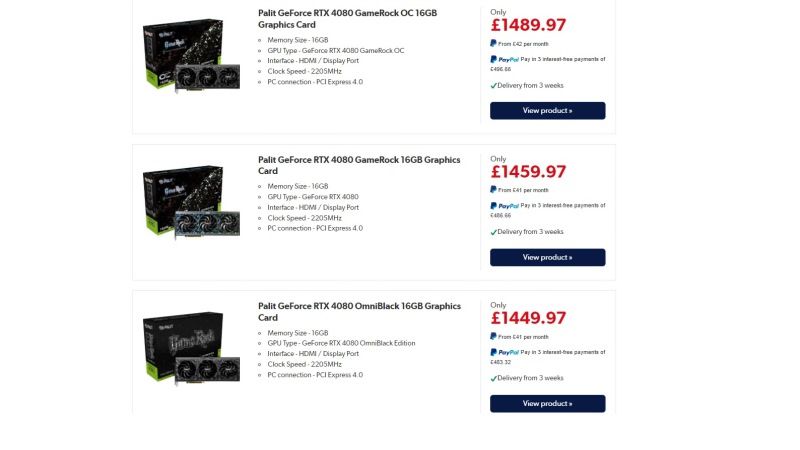The image showcases a Pallet GeForce RTX 4080 GAMER KOC 16GB graphics card prominently displayed on the left. The box is sleek and modern, with the model name clearly visible. Key specifications listed below the box include a memory size of 16GB and a clock speed of 2205MHz. The graphics card features an HDMI/DisplayPort interface and connects via PCIe 4.0. 

Highlighted pricing details show it costs 1,499 Euros, with an option for installment payments of $42 per month through PayPal, with the option to Pay in 3 interest-free payments denoted by a checkmark. The product is delivered through a service called Wings, and a "View Product" link is available for additional details.

Several repeating sections underline the same information: the graphics card’s model, memory size, and technical specifications. The price appears again, slightly varied at 1,459.97 Euros and 1,449.97 Euros in different sections. 

On the far left, the box features an image with an OmniBlack color theme, sectioned and bordered to structure the advertisement layout neatly.